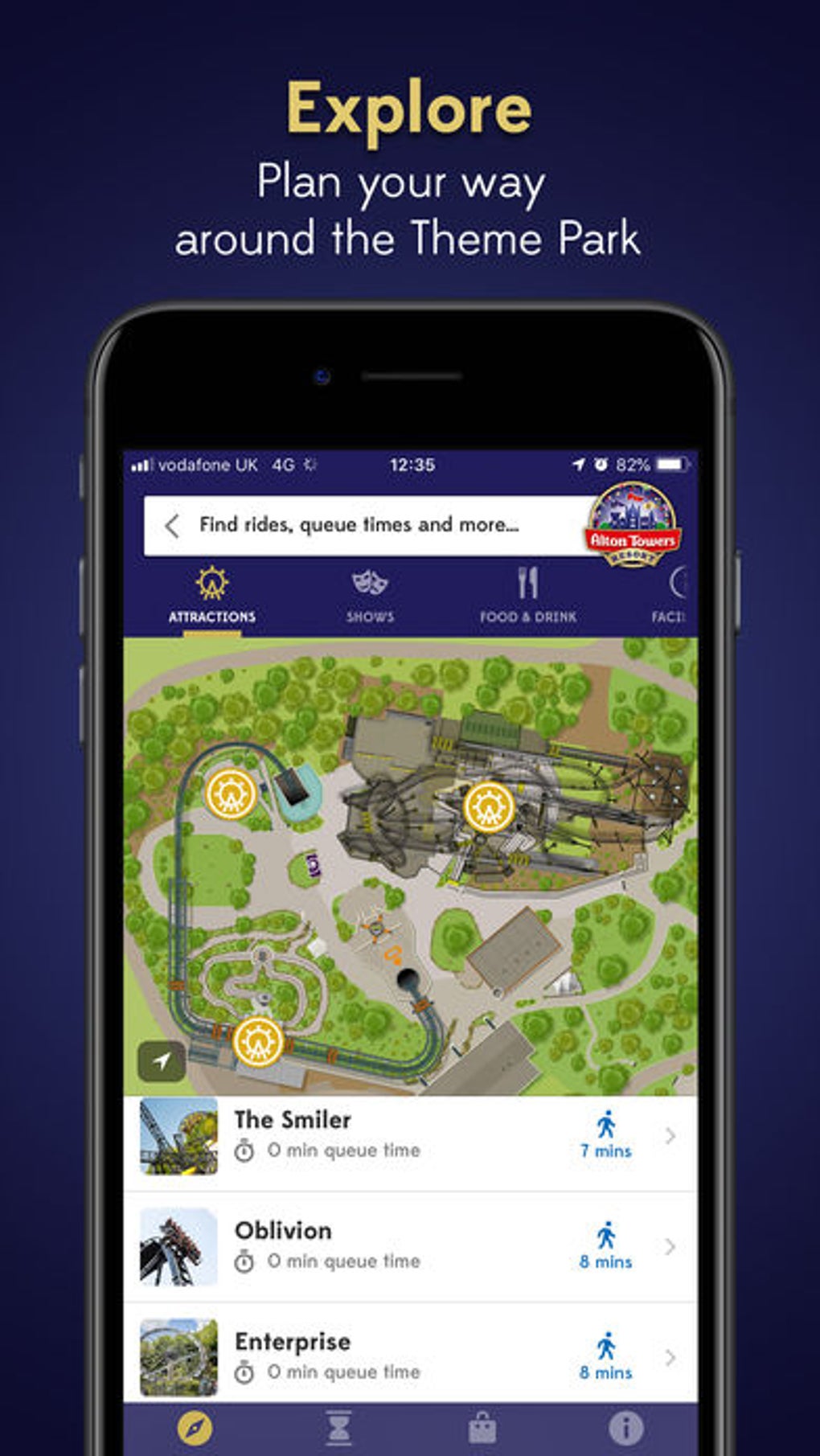Here's the cleaned-up and detailed caption for the image:

---

The image resembles a sleek advertisement that could be encountered online or on a billboard. It features a background with a dark blue hue, enhanced with a tastefully done vignette effect. Dominating the advertisement is a bold, yellowish-gold heading proclaiming, "Explore," which encourages viewers to "Plan your way around the theme park." Below the heading, a detailed mobile phone interface is prominently displayed.

The phone screen shows a detailed map of Alton Towers Theme Park, clearly positioning this scene in the UK, as indicated by the Vodafone UK 4G network icon, and the time displayed is 12:35 with 82% battery remaining. At the top of the screen, a white search bar invites users to "Find rides, queue times, and more."

Beneath the search bar is the Alton Towers Resort logo, followed by categorized navigation buttons labeled "Attractions," "Shows," "Food & Drink," and "Facts," each depicted with relevant icons like a Ferris wheel for attractions. 

The map below the categories highlights various popular rides, including The Smiler, Oblivion, and Enterprise, along with estimated walking times to each ride. The overall design conveys an intuitive and user-friendly mobile experience, making it clear that the application is designed to help visitors navigate and maximize their enjoyment of the theme park.

---